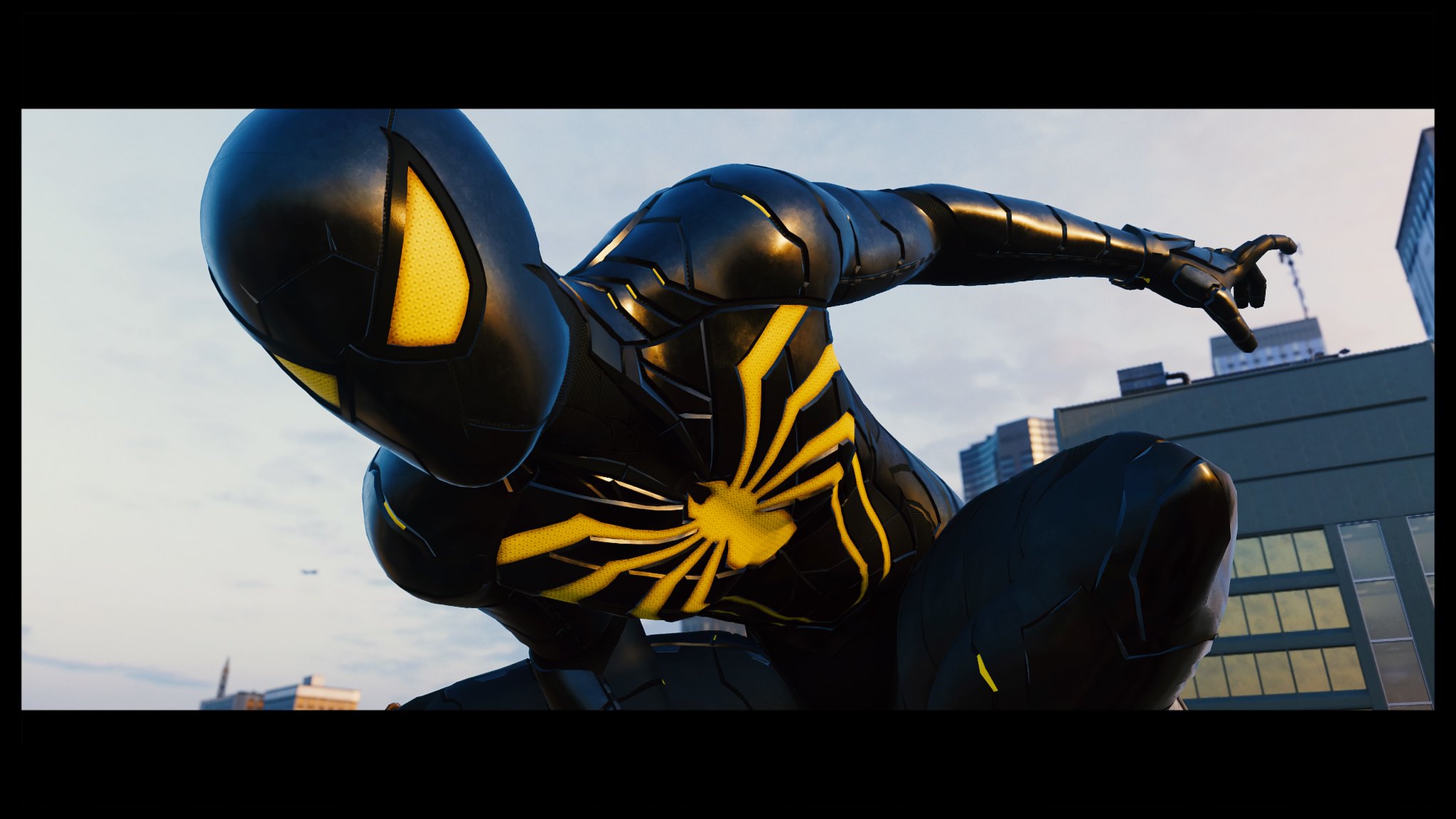In this striking image, Spider-Man is depicted wearing his iconic black suit against a backdrop of a cloudy, overcast sky. Positioned dynamically above the camera, Spider-Man appears to be readying himself for action. His left hand is poised to sling a web, with his fingers forming the familiar web-shooting gesture. His suit, a sleek black design, includes a leather mask with plain white eye lenses, giving him an enigmatic look. Prominently displayed on his chest is a white spider emblem, its eight legs sharply contrasted against the black fabric. The bottom two legs of the spider integrate into web-like designs that extend downward.

Behind Spider-Man, to the left, stands a modern office building characterized by its gray, likely metallic, upper structure and at least three stories. The unusual angle from which the photo is taken—almost from ground level—creates an optical illusion, making the building appear as though it is emerging from Spider-Man’s hand. Spider-Man's left leg is bent at the knee, adding a sense of motion and readiness, while his right arm is hidden from view, enhancing the dramatic tension of the scene. The overall composition captures a moment brimming with potential energy, set against an urban backdrop that enhances the superhero's presence.